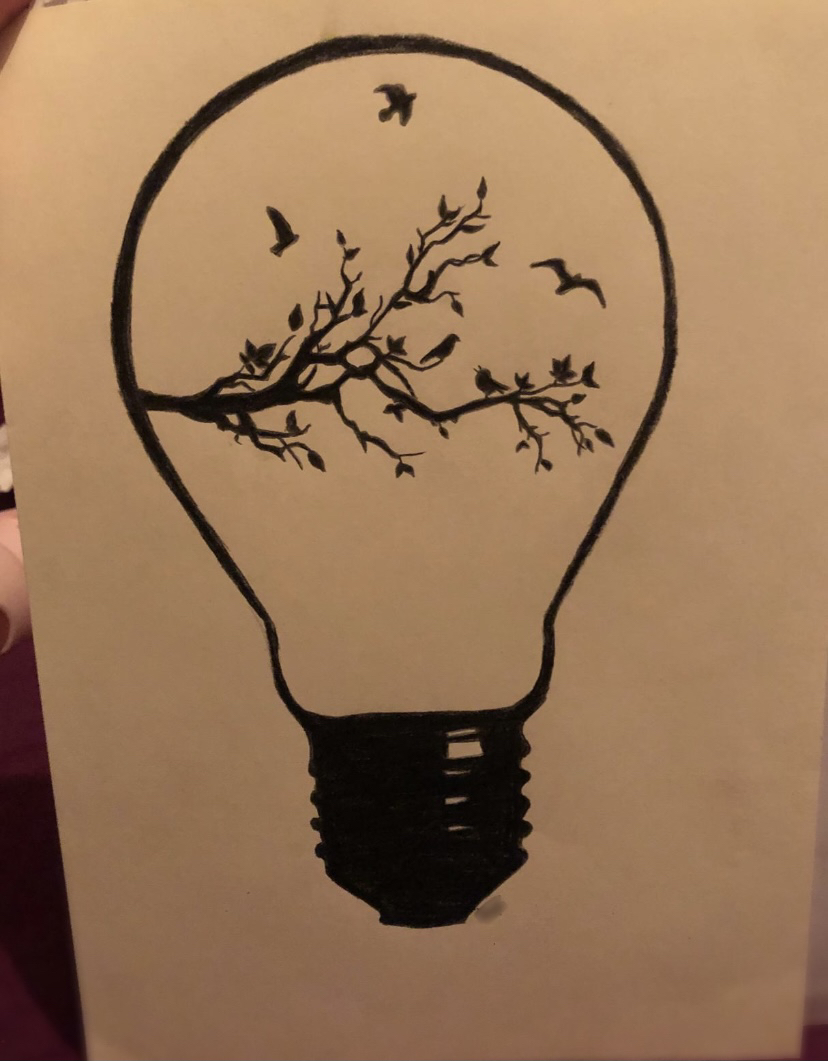This detailed artwork features a striking depiction of a lightbulb at its center, set against a stark white background. The lightbulb, outlined in bold black, has a circular upper half that transitions into a solid black base. Intriguingly, the interior of the lightbulb is filled with a monochromatic scene of birds and branches. Birds can be seen both flying and perching, with one prominent branch extending from the left side, adorned with subtly detailed leaves. The entire image maintains a black-and-white motif, enhancing its dramatic visual impact. In the bottom left corner, there appears to be a faint, indistinct element in the background, adding a layer of mystery to the composition.